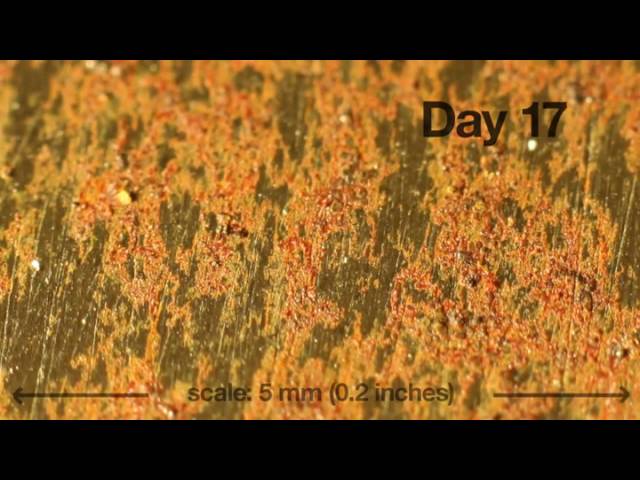In this image, we see a detailed close-up of a textured platform featuring a blend of orange, red, yellow, and green hues, with noticeable vertical striations. The surface is punctuated by bright white specks resembling tiny crystals, predominantly visible in the middle left area and extending across the top. The overall composition is set against a backdrop that appears to mimic a natural landscape, perhaps reminiscent of a greenish, dark earth.

The platform is bordered by thick black bezels on the top and bottom, similar to a frame from a film reel. In the upper right corner, the bold black text "Day 17" or "Gage 17" is prominently displayed. At the bottom center, a precise scale is indicated with the text "scale: 5 millimeters (0.2 inches)" in a small black font, flanked by thin black arrows pointing outward to the left and right. The detailed and varied coloration and texture of the platform, combined with the precise annotations, create a striking and informative visual presentation.